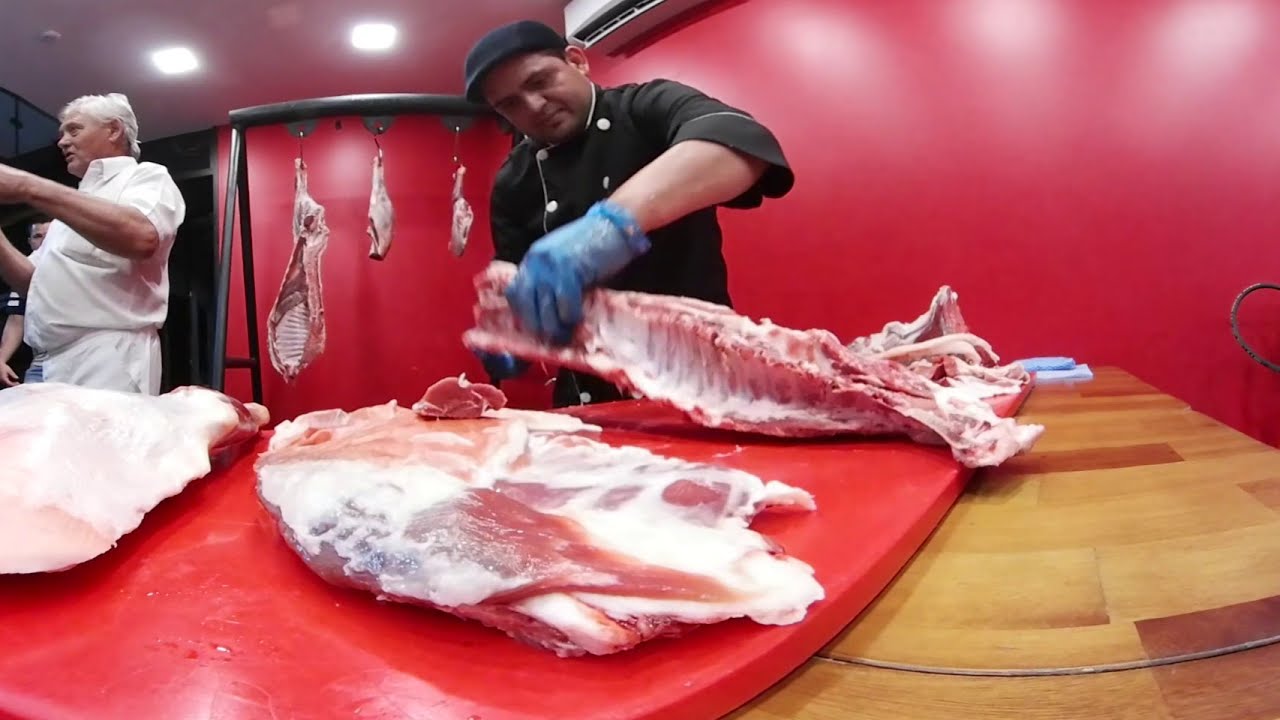In an indoor butcher shop with recessed lighting from above, two men are diligently preparing meat on a rich wood countertop adorned with a vivid red cutting board. Centered in the scene, a butcher in a black uniform with white buttons and a matching black ball cap meticulously handles a slab of marbled meat with his blue-gloved hands. To the left, another butcher dressed entirely in white, with gray hair, engages in conversation, suggesting interaction with a customer or colleague. Behind them, the vibrant red walls of the shop are lined with hooks, from which various pieces of meat hang. The atmosphere is bustling and focused, captured in the midst of the butchering process.